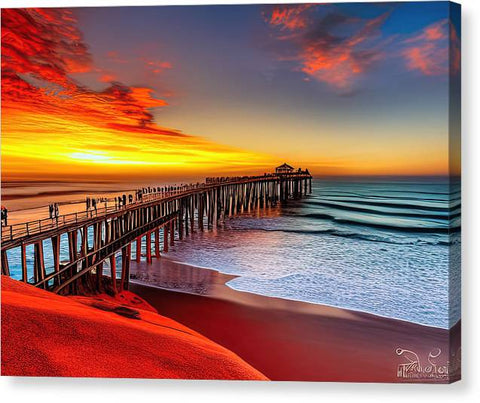The image portrays a striking scene of a wooden fishing pier extending into the ocean, captured as a vibrant, touched-up photograph printed on a wrapped canvas, where the artwork continues around the edges. The pier, set on stilts and lined with walkers and fishermen, culminates in a pergola-type structure at its end. The dramatic sunset bathes the scene in a symphony of colors, with the upper left sky showcasing radiant, illuminated clouds in bright yellows and oranges, while the upper right transitions to a darker blue with tinges of orange highlights. Below, the water gently laps at the shore, creating a foamy white edge against the wet reddish-gold sand, reminiscent of Australian dunes. In the foreground, these dunes provide a textured contrast to the blue waves further in the distance. The canvas is signed in the bottom right corner in a white script, adding a final personal touch to the warm, dynamic composition.